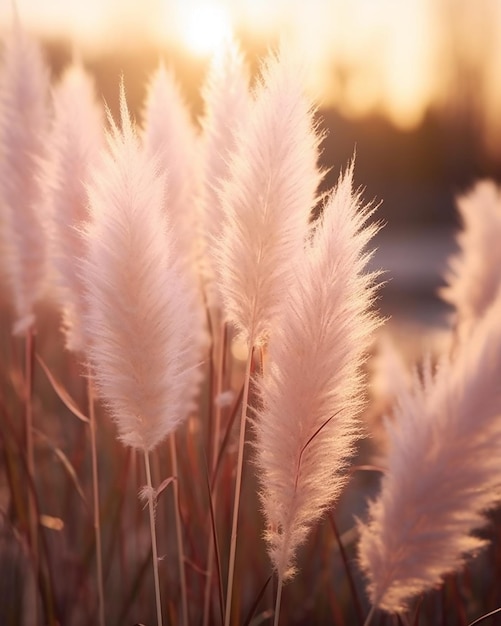This is a close-up photograph of wispy, feather-like plants captured in fine detail in the foreground. The plants exhibit long, narrow stems that range from light brown to a pale, almost white, tan color. Their tops feature elongated, fluffy, pointed oval shapes that resemble delicate feathers or animal tails, adding a sense of movement as they extend in various directions. These feathery plumes are predominantly light-colored, with shades of white and very light brown. The composition shows about eight or nine of these plants cascading diagonally from the upper left to the lower right of the image. The foremost plants are crisply in focus, while those further back become progressively blurrier, enhancing the depth of field. The background, enveloped in a soft, pale golden hue transitioning to darker brown shades, is out of focus, hinting at potential water, trees, or buildings bathed in sunlight, yet remaining indistinct. This golden backdrop, combined with blurred dark tones, suggests an outdoor setting bathed in warm light, further highlighting the ethereal quality of the plants.